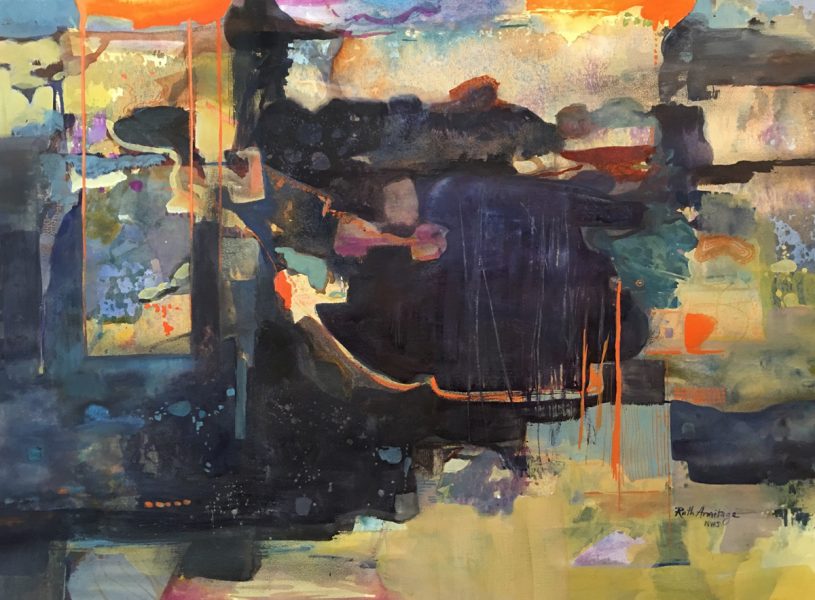This image is a scan of a horizontal rectangular abstract painting, approximately one and a half times as wide as it is tall. Dominated by bold and varied colors, the composition centers around an interplay of blues, dark purple, and black, suggestive of water. Surrounding this central area, especially on the left, top, and right, is a vibrant mix of oranges, beiges, and lighter blues. Adding to the dynamic palette, there are splashes of pink, orange, gray, blue-green, and blotches of yellowish-green at the bottom right. The painting also features areas where orange paint appears to drip down, creating an impression of multiple suns at the top left and right. The central part of the artwork includes a brown stroke that could be interpreted as a boat in the water. There is a suggestion of a landscape at the bottom of the image, depicting more land in shades of orange-yellow-beige. Additionally, the painting bears a signature that reads "Ruth Armitage." Overall, the stylistic elements and color dynamics make this piece suitable for display in an art show, inviting viewers to use their imagination to discern its abstract elements.